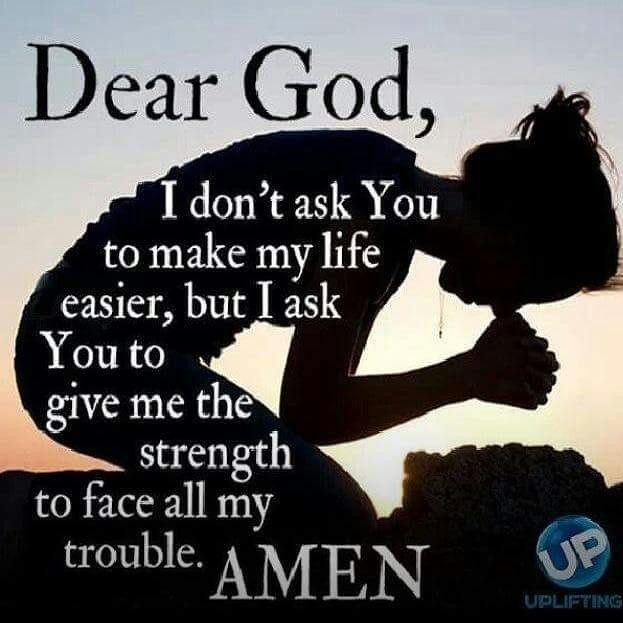The image is a square-format, color photograph featuring the silhouette of a kneeling girl with her hands brought to her face in a prayer-like position. The background showcases a gradient sunset, transitioning from pale orange at the bottom to a deep blue at the top. Overlaid on the silhouette, which is in complete black, is inspirational text in white letters that reads: "Dear God, I don't ask you to make my life easier, but I ask you to give me the strength to face all my trouble. Amen." The words "Dear God" are in black. A minimalist necklace is faintly visible around the girl's neck. In the bottom right corner, there is a blue circle logo with the word "UP" in bold white letters at an angle, and beneath it, the word "uplifting" in blue text. The image blends photographic representationalism with typography and graphic design, creating an inspirational or religious meme-like piece.